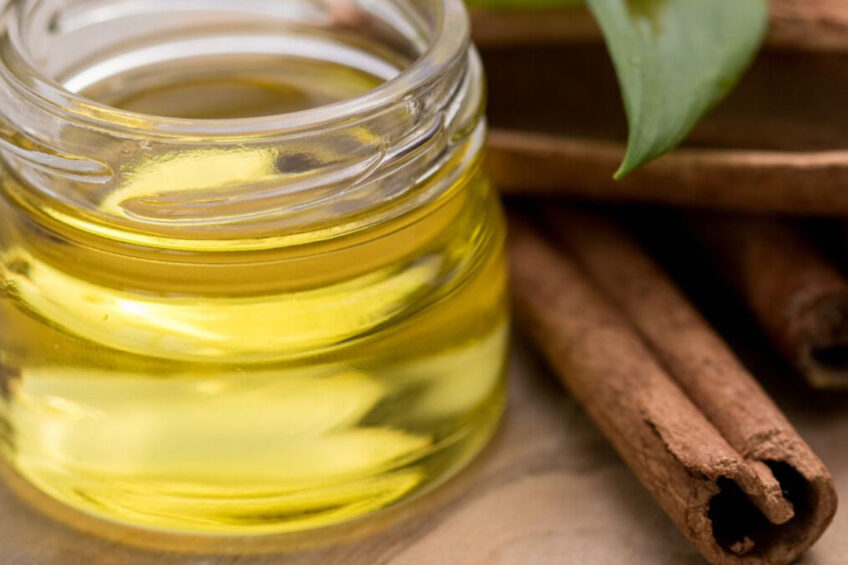In this close-up image, you see a clear glass jar filled almost to the brim with a bright yellow liquid, possibly honey or oil, resting on a light brown, somewhat misshapen wooden surface. To the right of the jar, you find a large cinnamon stick in sharp detail and, slightly further back, a smaller cinnamon stick. The top right corner of the image features a vibrant green leaf hanging down. The background and bottom part of the image appear blurry, with a nondescript brown object above the cinnamon sticks and another object resembling a ball. The jar lacks a lid and has about a half-inch of space left unfilled at the top, giving the scene a clean and organized look against its natural, rustic backdrop.